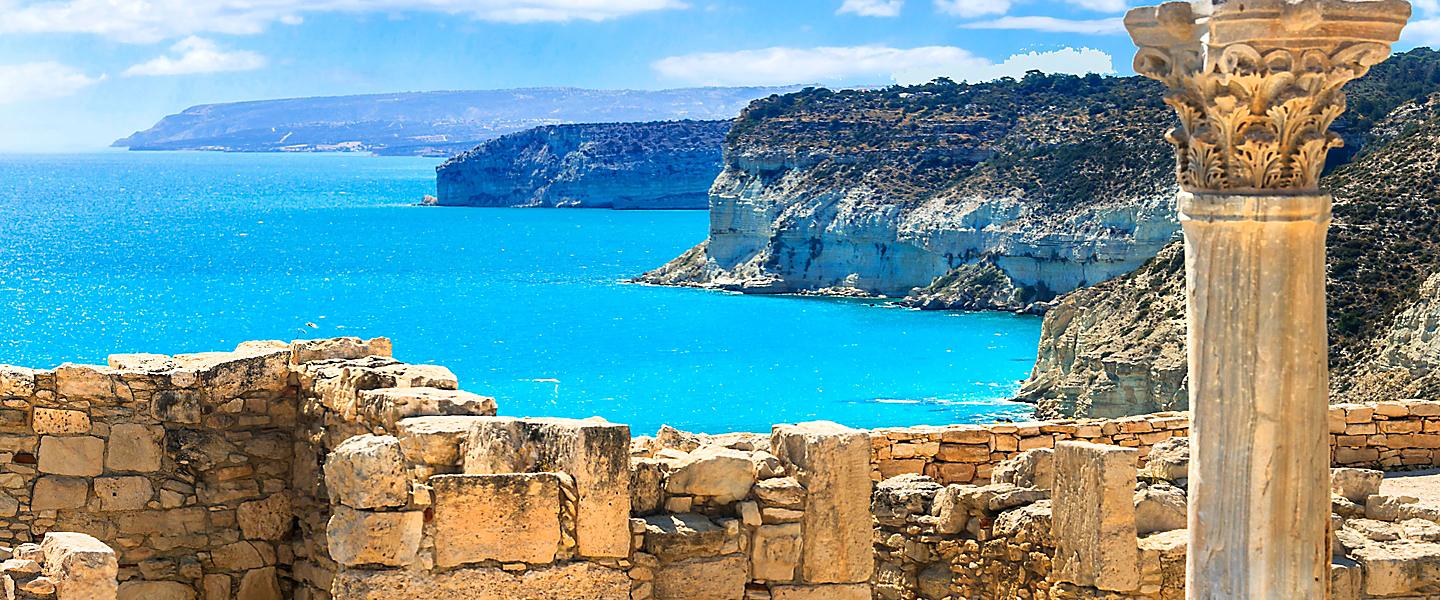This photograph captures a stunning coastal scene bathed in brilliant sunlight. In the foreground, there is a crumbling, ancient rock wall with stones of various shapes and sizes arranged in a distinctive zigzag pattern. Adjacent to the wall on the right is an ornately carved stone column, featuring intricate leaf-like designs at its top, further indicating its age and historical significance. The immediate background reveals steep, rocky mountains with sparse vegetation, such as brown, dead grass and smaller rocks clinging precariously to the edges. These rugged cliffs lead directly into the strikingly turquoise blue ocean, which mirrors the equally vibrant blue sky adorned with fluffy white clouds. Beyond the initial coastline, a small rocky peninsula juts out into the sea, adding depth to this picturesque landscape.